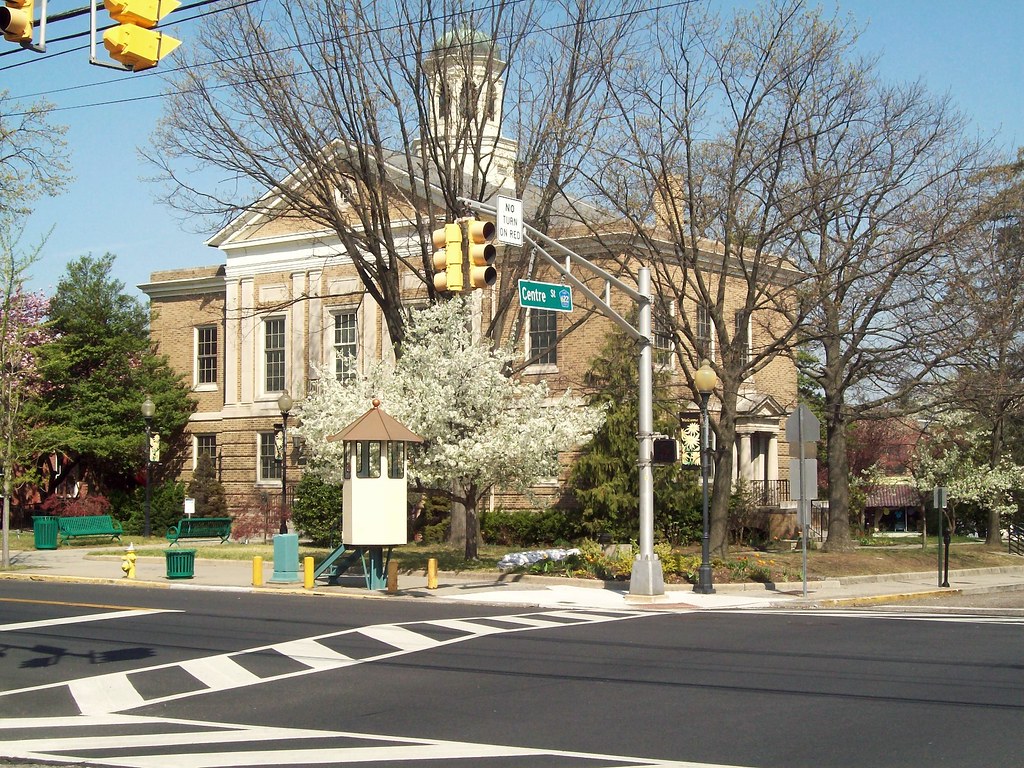This full-color photograph captures a clear winter or early spring day, focusing on a street corner intersection at Center Street. The lower part of the square image prominently features a paved street with freshly laid blacktop, clearly marked with a white crosswalk and a yellow dividing line. A gray traffic light pole stands at the intersection, supporting a yellow lamppost and a green street sign that reads "Center Street." Another sign indicates "No Turn on Red."

Behind the intersection, a large, two to three-story brick building dominates the scene. This building, which might serve as a library or public facility, boasts a tan stone exterior with several grid-pattern windows. Notably, the building also features a rooftop tower with a rounded design and windows. Surrounding the building is a mix of tall hardwood trees devoid of leaves and a few pine trees, with one smaller tree covered in white foliage. The sky overhead is a crisp, clear blue, adding to the overall serene yet stark winter ambiance.